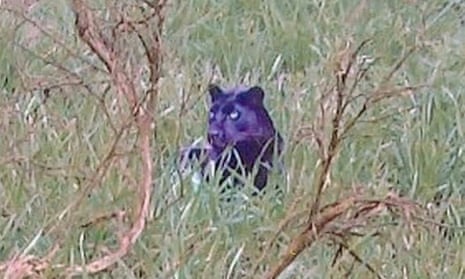A black panther stands concealed in very tall, shiny grass that reaches up to its neck, obscuring its legs and much of its body. The panther's sleek black fur and almost glowing green eyes are prominently visible as it looks slightly up and to its right. The image, likely taken from a distance with significant zoom, appears to be of lower quality, suggesting the photographer intended to stay concealed. The scene is set during the daytime; there is adequate lighting, although it could be slightly overcast. Surrounding the panther are tall, thick green grass blades and a few brown, leafless branches in the foreground, adding to the sense of a wild and natural habitat. The panther’s pointed, upright ears and its positioning suggest it might be lying in wait, possibly for prey.